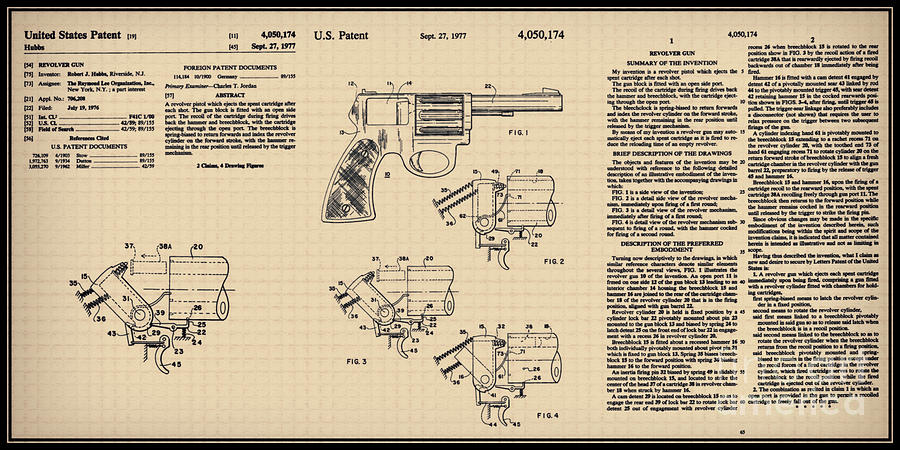The black-and-white horizontal image features a yellowed, aged piece of paper with a black border around the entire page, giving it an antiquated appearance. In the upper left-hand corner, the words "United States Patent" are prominently displayed alongside small text and numbers indicating page numbers and references to foreign patent documents, though these details are quite small and hard to read. The focal point of the image is a detailed, labeled drawing of a revolver, showcasing all the various parts such as the barrel. There are multiple figures on the page, with figure one displaying the gun, and figures two, three, and four illustrating potentially the inner workings of the revolver. To the right of the gun illustration, the page is divided into two columns containing several paragraphs of text. These sections include the "Summary of the Invention" and "Description of the Preferred Embodiment," offering detailed written information about the revolver.